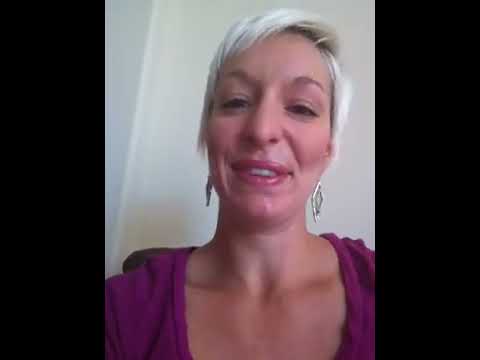The image is a close-up, square photograph with thick vertical black borders on each side, focusing on a middle-aged, light-skinned woman with short blondish-white, or possibly silver-gray, colored hair parted to the left. She is smiling widely, revealing her top teeth, and is adorned with large diamond-shaped, silver earrings. She is wearing dark pink lipstick, which complements her well-defined eyebrows, and a purple top with a drooping neckline that leaves her chest and shoulders exposed. The background is a plain white wall with a hint of a black chair just visible at the bottom, suggesting an indoor setting. The overall look and setup give the impression that this could be a selfie, possibly taken for social media.